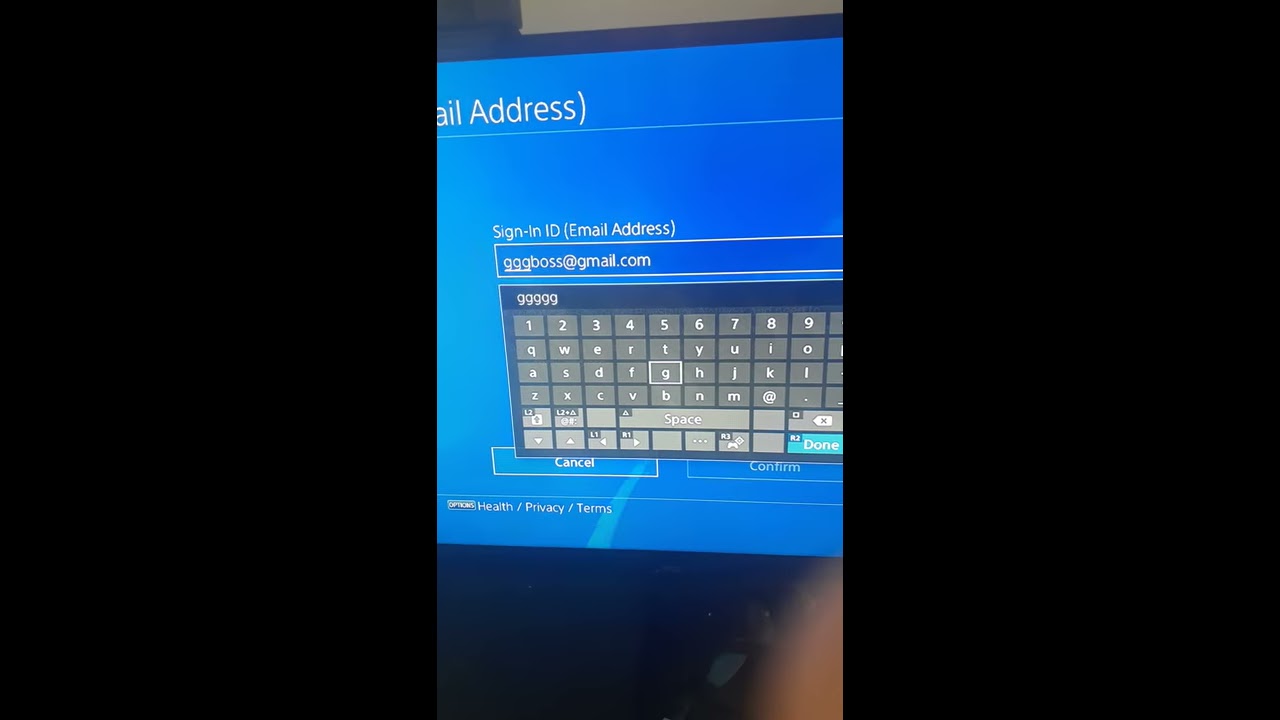This image captures a photograph of a computer or television screen displaying a sign-in page, most likely for the PlayStation Network. The screen features a blue background with a virtual keyboard overlaid. At the top, the text reads "email address" and "sign in ID (email address)," partially cut off to show only "AIL address." Below, the email address "gggboss@gmail.com" is entered. Options for "cancel" and "confirm" are visible beneath the entry field. Further down, the screen displays the terms "health," "privacy," and "terms." The screen occupies the central third of the image, flanked by black rectangles on either side, with some indistinct background details possibly showing the room's wall. The photograph appears to be a reminder or a documentation of the sign-in process.